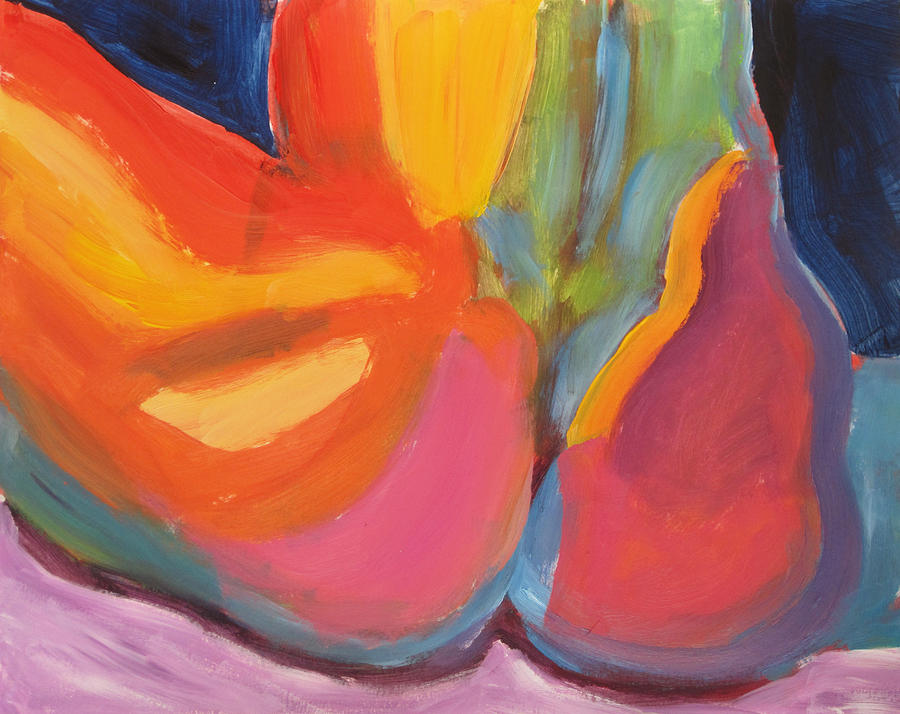This vibrant, square abstract painting is a spectacular display of colors and brushwork, without any definitive borders or background. The bottom portion is dominated by a soft purple hue, providing a contrast to the more intense colors above. The upper left and right corners are primarily dark with black brushstrokes, but the center bursts with a multitude of vibrant colors, including reds, yellows, blues, and greens. These colors intermingle beautifully—yellows blend with blues to create greens, and yellows with reds to produce oranges. Amidst this colorful chaos, there appears to be a peach-centered orange circle and various abstract, broken triangles in blue, orange, and yellow. Additionally, the right side features a red pattern resembling a pear, surrounded by blues and yellows. On the left side, there's a pink, inverted crescent moon-like shape next to an abstract form combining orange and yellow hues. Throughout the painting, other colors such as pink, cream, and light green contribute to the overall richness, making it an intense, vivid expression of abstract art.